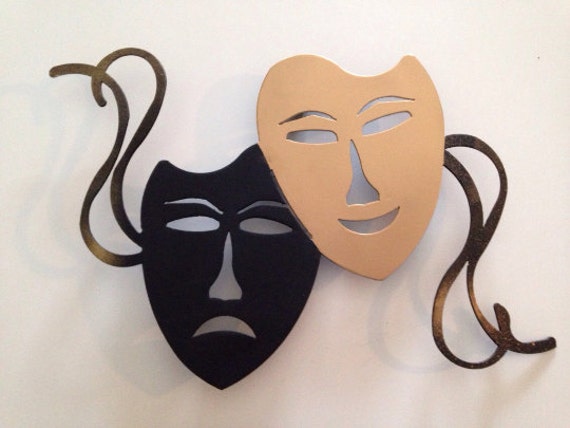The image showcases two theatrical masks positioned against an off-white, cream-colored background in landscape mode. The left mask, painted black and with a thick, velvety appearance, represents tragedy. It features cutouts for the eyebrows, almond-shaped eyes, nose, and a deeply downturned frowning mouth. To the right of it and slightly above, there is a beige (light cream/tan) comedy mask. Similar in design, this mask has rounded rectangular cutouts for the eyes, arched eyebrows, and a nose, but with an upturned, smiling crescent mouth. Both masks are adorned with brown, leather-like or possibly metallic spiraling ties, suggesting they are intended to be worn, with the black mask's strings stretching towards the upper left corner and the beige mask's strings extending towards the bottom right corner. Together, they cast light shadows against the background.